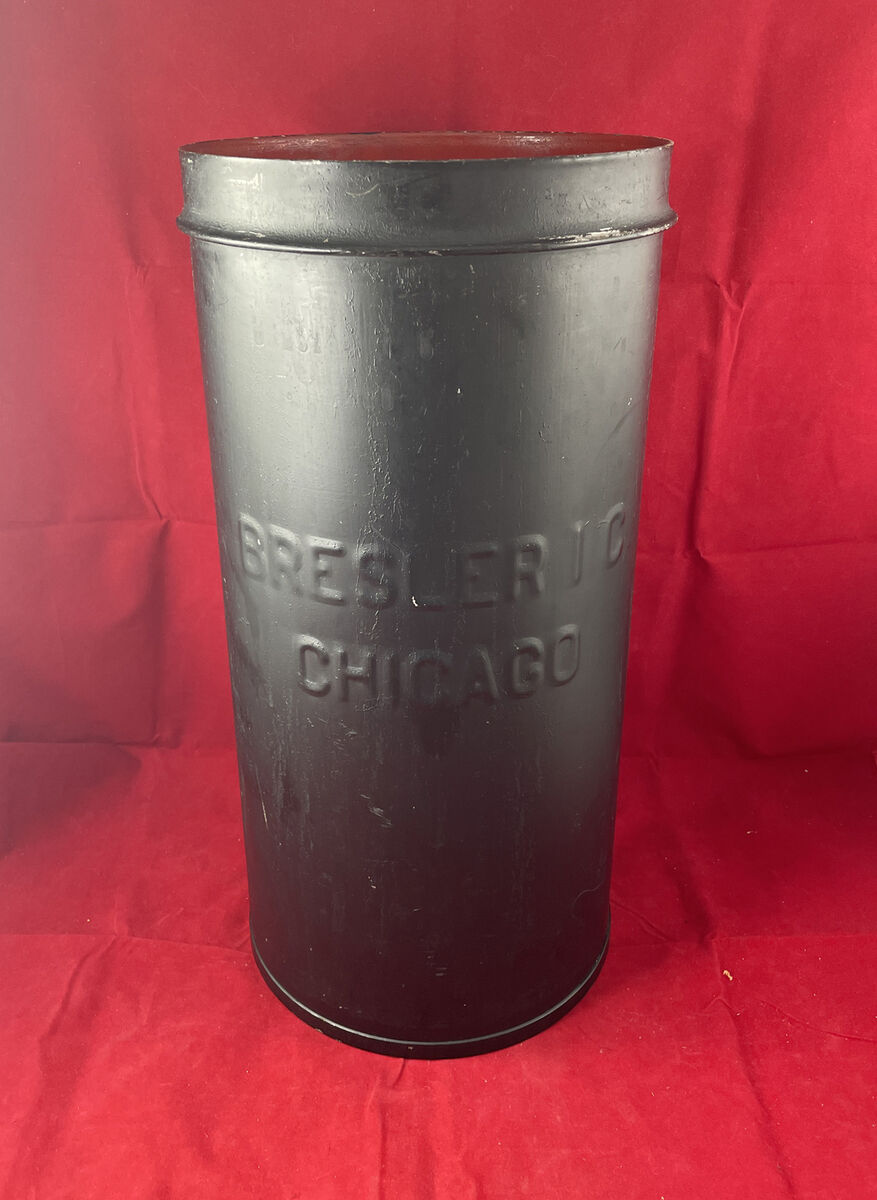The image features a very old, vintage container made of dark gunmetal, characterized by its unpainted, natural gray color that reveals wear and tear over the years. The cylindrical container, which may slightly taper off like a steeply sloped cone, stands upright on a red surface that matches the backdrop, suggesting it could be a red tarp, sheet, or upholstery. The container is adorned with raised, embossed lettering that reads "Bressler 1C Chicago," indicating its origin. Its metal lid appears tightly sealed on top. The container exhibits signs of age such as chipping, dirt spots, and a few dents. The red background and surface create a striking contrast, and the image provides a close-up view, revealing light reflections at the top edges of the container.